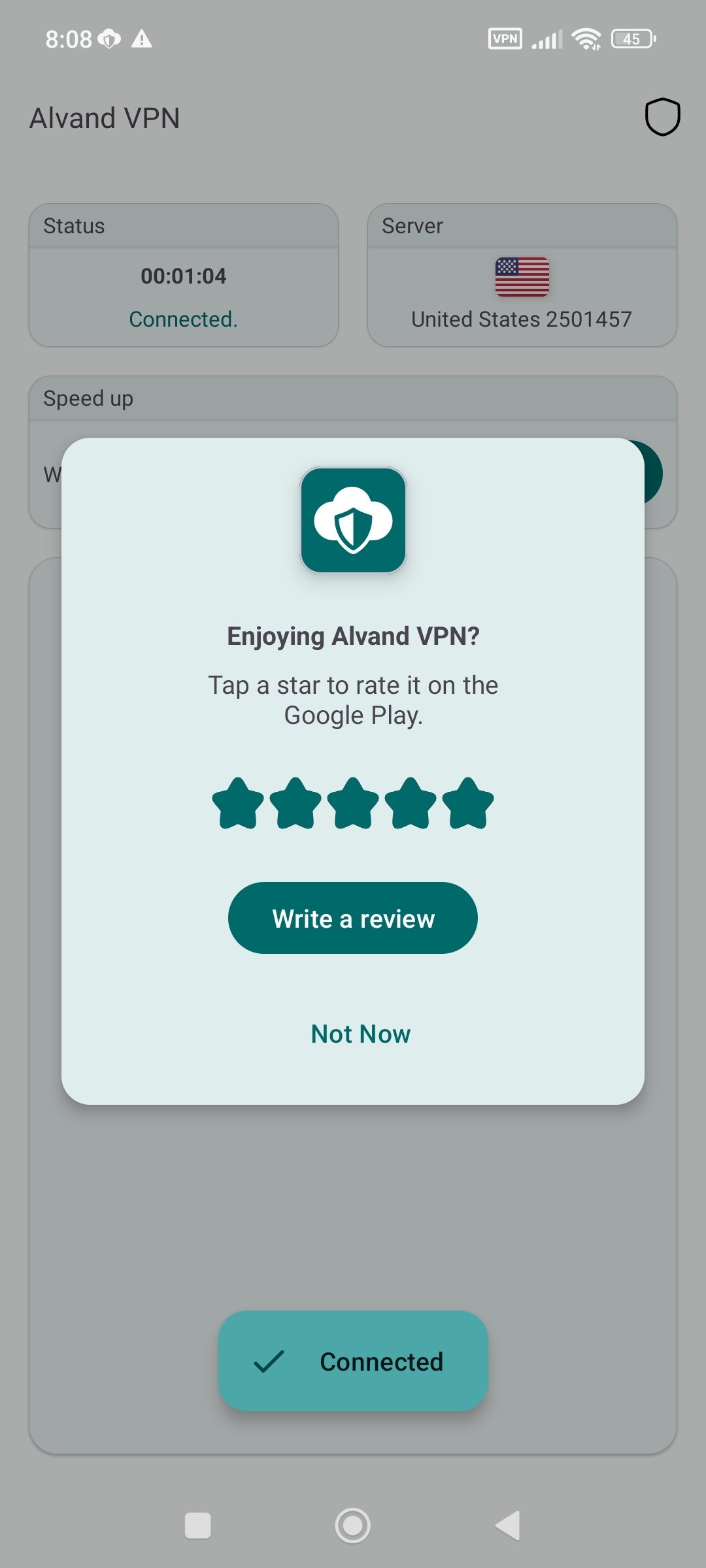This image is a cell phone screenshot displaying the interface of an application at 8:08, as indicated in the top left corner. The top right corner shows the battery at 45% charge. Central to the screenshot is a pop-up window prompting a review for the Avalan VPN app. The window reads, "Enjoin Avalan VPN. Tap a star to rate it on Google Play," and includes five dark turquoise stars for rating. Below the stars, there are two options: a "Write a Review" button and a "Not Now" link.

In the background, the Avalan VPN application interface is visible. It shows the current server located in the United States and indicates an active connection that has lasted one minute and four seconds. At the bottom of the screen, a blue teal-colored button labeled "Connect" with a checkmark on its left confirms the connection status.